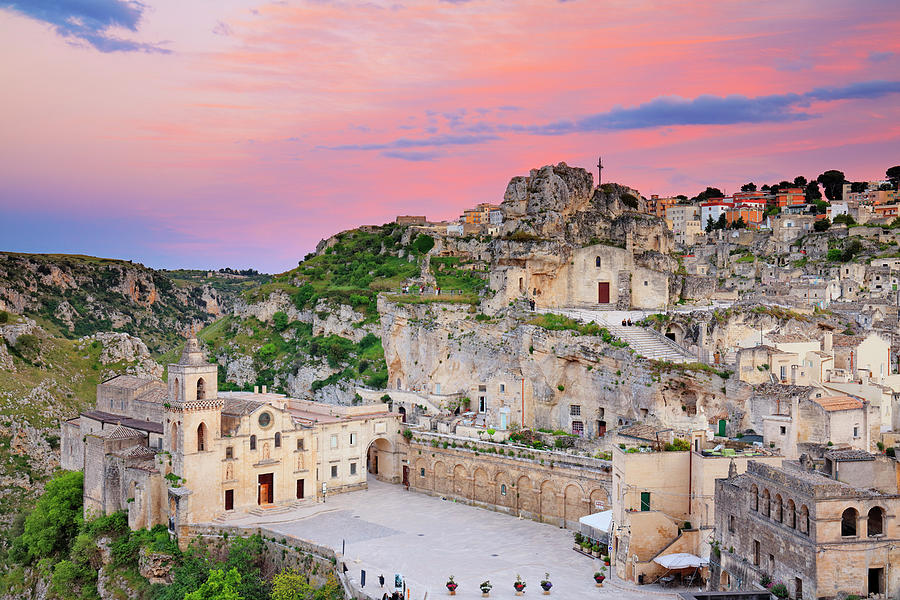The image depicts a picturesque hillside village, reminiscent of an ancient European or Mediterranean town, with a possibility of it being in Israel or Italy. The professionally-captured photo showcases an array of old, white, and terracotta stone buildings that appear to be crumbling yet exude historical charm. Nestled among rocky cliffs and mountainous terrain speckled with green shrubbery and trees, the village gives the impression of structures carved directly into the rock. Archways, patios, and fences accentuate the scene, while in the foreground, a large wall divides two sections of the village. The lower courtyard area features blue and red objects that could be pots with plants, adding a dash of color. Some buildings have red doors and steeples, suggesting their use as churches. The sky overhead is a stunning palette of pink, blue, white, and a hint of purple, evoking either sunrise or sunset with its fluffy clouds. This vivid and tranquil setting lacks any text, people, or animals, leaving viewers to marvel at its untouched beauty.